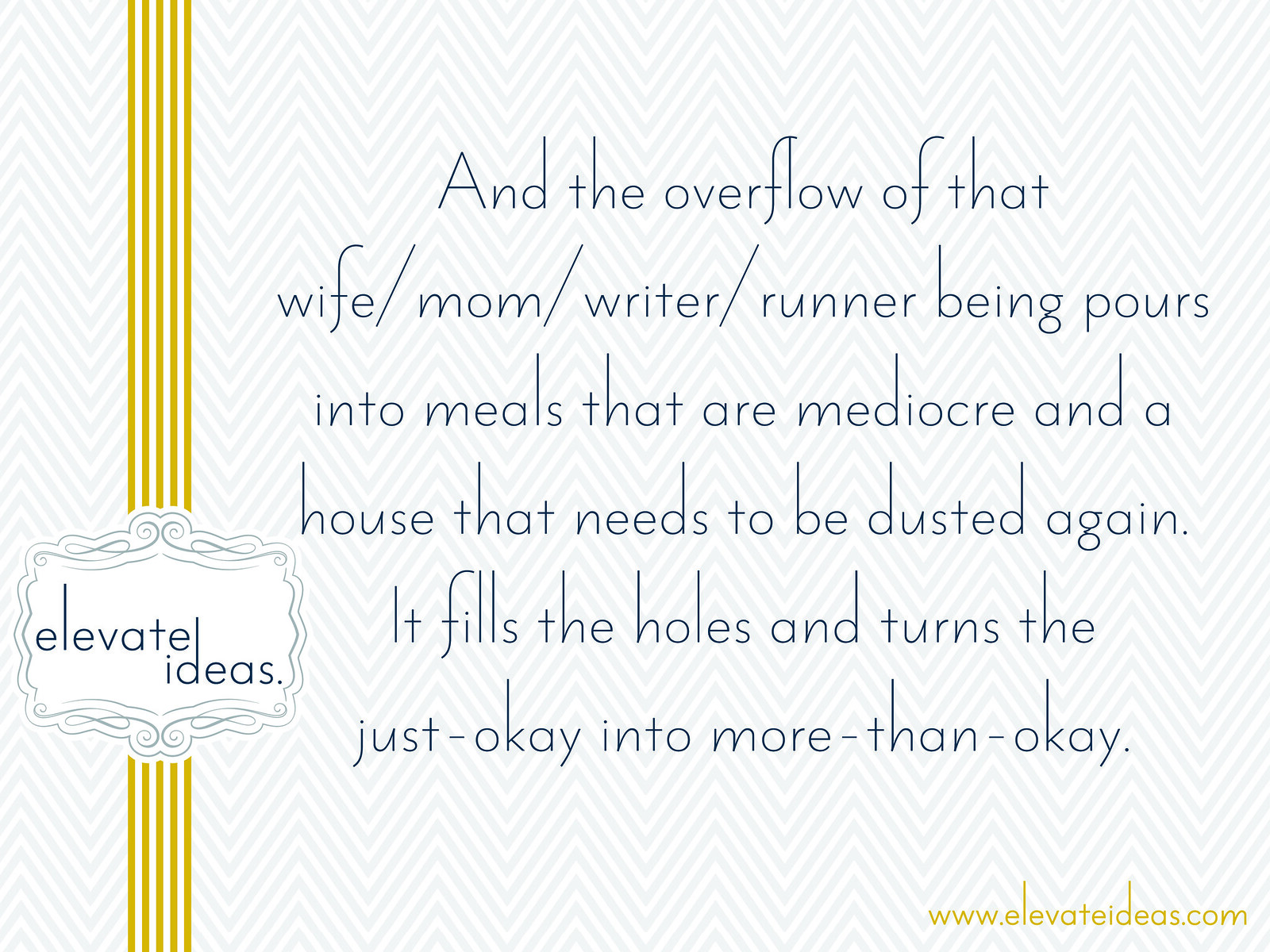The large square image features a background with light blue, zigzagging lines that alternate with white, creating a chevron pattern. On the left side, five vertical lines in a yellowish-brown hue run from top to bottom. Positioned across these vertical lines is a decorative badge-like rectangle with curvy edges containing the text "Elevate Ideas." Dominating the right side of the image is a detailed motivational message written in blue: "And the overflow of that wife/mom/writer/runner being pours into meals that are mediocre and a house that needs to be dusted again. It fills the holes and turns the just okay into more than okay." In the lower right-hand corner, the website "www.elevateideas.com" is inscribed in yellowish-brown letters. This image appears to be a promotional flyer designed to inspire, with an emphasis on personal growth and creativity.